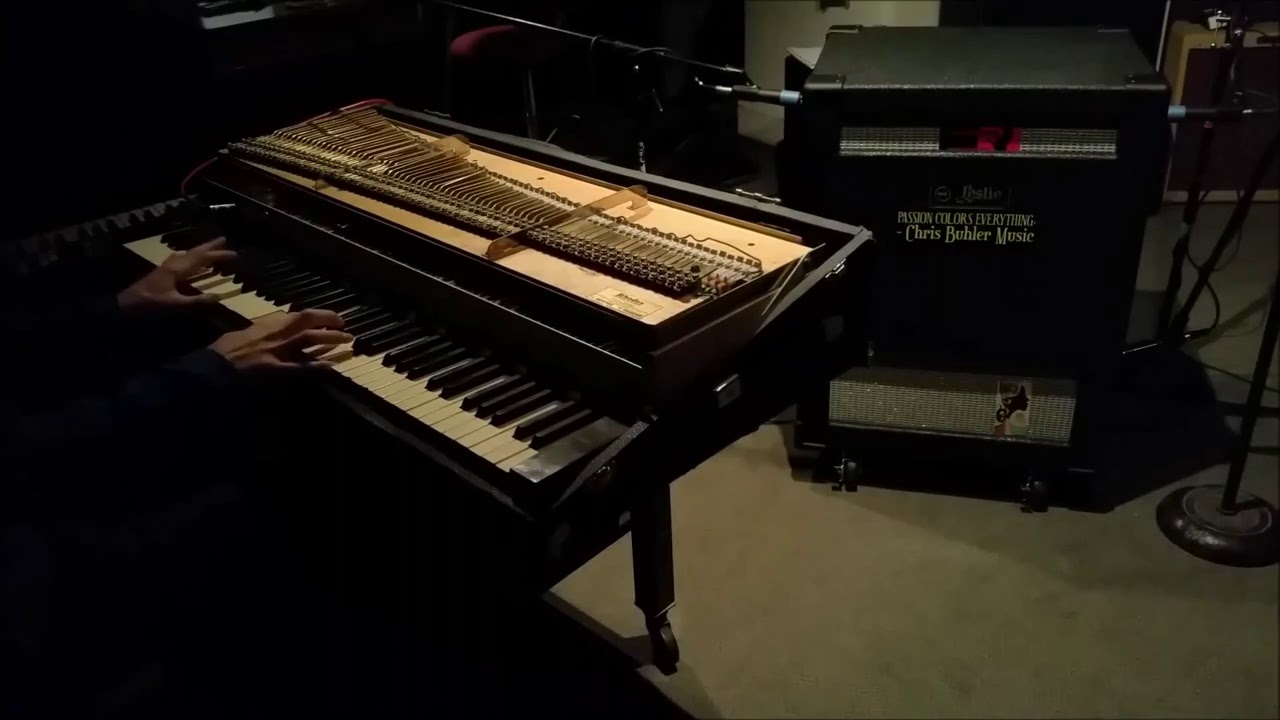In this shadowy image, two disembodied hands emerge from the darkness to play a small, black piano with its top open, revealing the intricate inner workings and strings. The full keyboard, featuring distinct black and white keys, is clearly visible. The hands, cut off at the elbows by the edge of the frame, stretch up and slightly to the right as they play. Below and to the sides of the piano, the scene fades into almost complete blackness, creating an eerie, floating effect for the hands. The floor, possibly pre-colored carpeting or a cement surface, is partially visible. In the background, assorted musical equipment is scattered, including a possible speaker, microphone stands, and a stand with rolling wheels displaying the name "Chris Buehler Music." Part of a white wall punctuates the scene, adding to the mysterious ambiance of the setting.